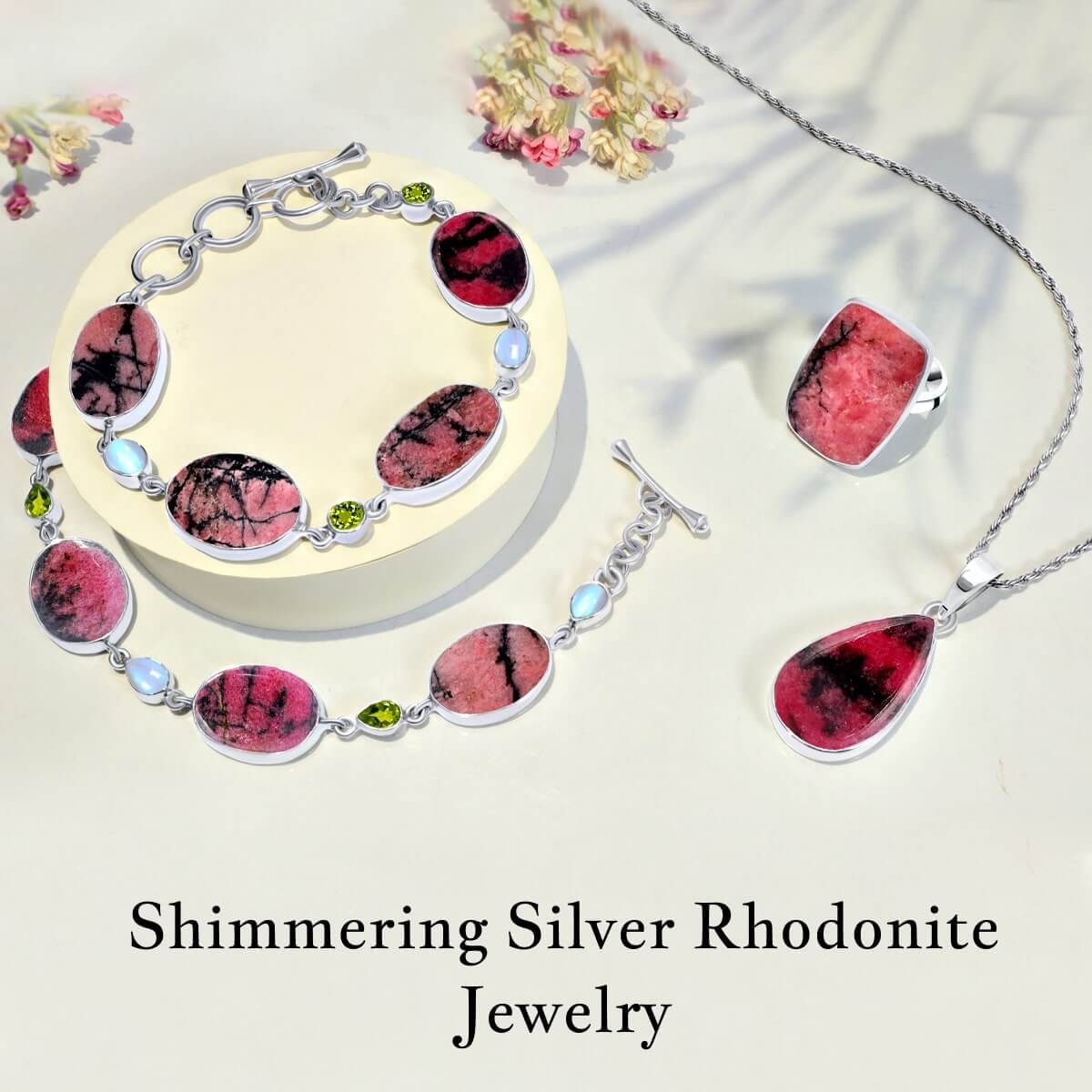The image showcases a matching jewelry set against a white background, prominently featuring silver chains and Rhodonite stones, characterized by their distinctive purply-red color interlaced with black, almost resembling marble or granite. The set includes a teardrop pendant necklace, a substantial cushion-cut ring, and two almost identical bracelets adorned with oval stones. Complementing the Rhodonite stones, the bracelets also feature smaller blue and green stones. Positioned on a white circular platform on the left, one bracelet showcases its design, while the other lies spread out with its clasp open. In the top right corner, shadows are visible, and the bottom of the image is labeled with black text reading, "Shimmering Silver Rhodonite Jewelry." Additionally, a few small red flower accents embellish the top and left sides of the composition, adding an extra touch of elegance.